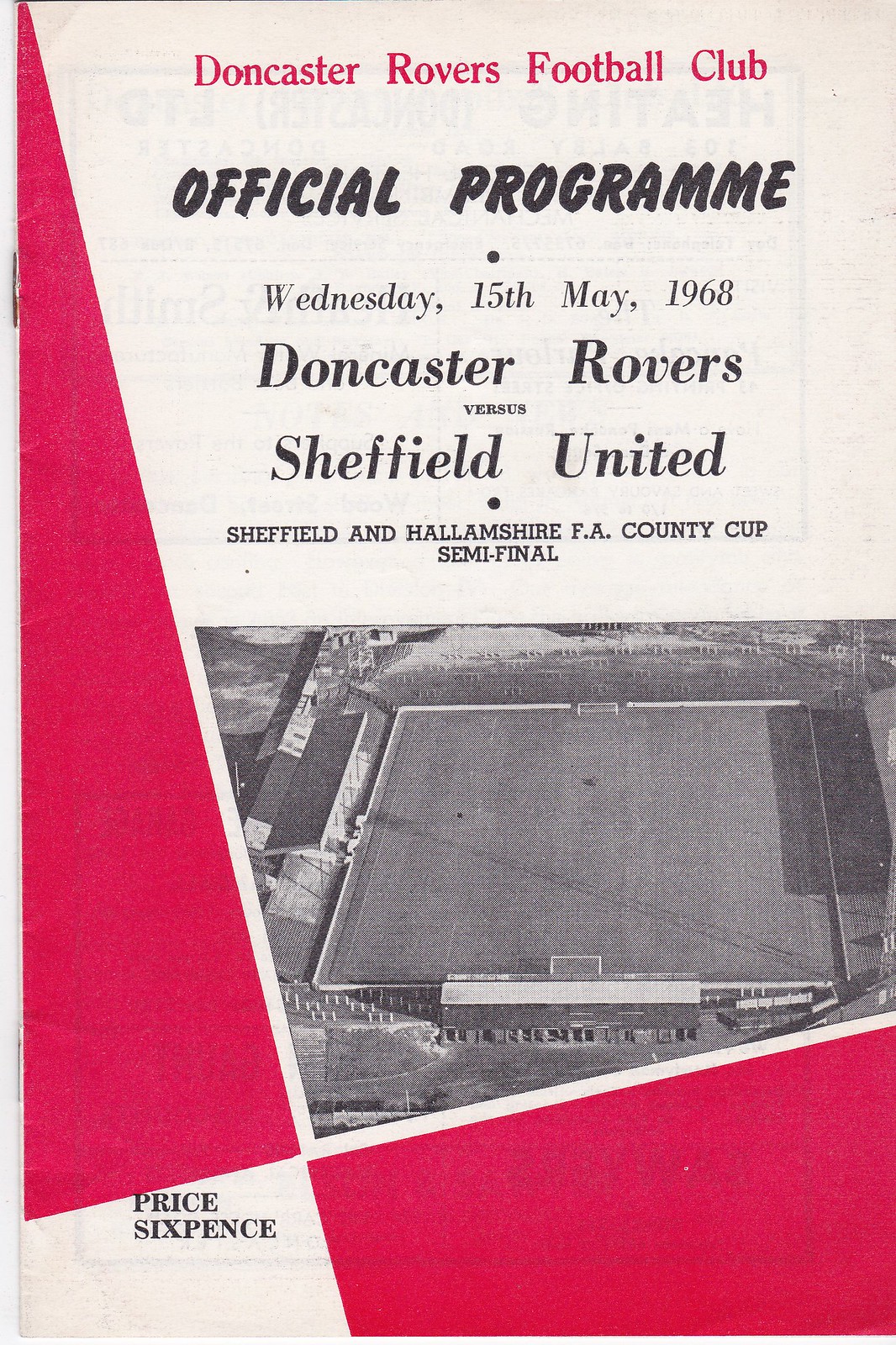This image features the front cover of an official program for the Doncaster Rovers Football Club. Dominantly white with intersecting red triangles along the left side and bottom right corner, it is titled in bold red letters at the top, "Doncaster Rovers Football Club". Below in black text, it reads "Official Program". The program is dated Wednesday, 15th May 1968, documenting a match between Doncaster Rovers and Sheffield United in the FA County Cup semi-final. At the bottom left, the price is indicated as six pence. Central to the cover is a black and white photograph of an empty football stadium, showing a field with goals at either end and no spectators or players visible, suggesting a bygone era. The design includes geometric patterns, adding an aesthetically retro touch reflective of its time.